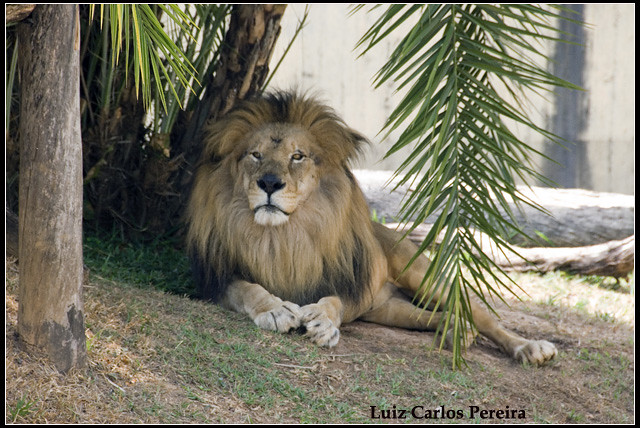The image captures a large male lion, prominently positioned in the center, sitting and resting on a short grassy area near a tree. This majestic lion, identifiable by his big, grayish-orange and black mane, has a distinctive black spot on his forehead and a relaxed demeanor. The scene suggests a warm, sunny day during summertime as sunlight illuminates the surroundings. The lion, exhibiting strong muscular legs and big feet, appears to be in good health and shade, indicating a peaceful moment.

Located in a zoo, the background reveals a large concrete wall, reinforcing the setting. Additional details include a large cylindrical tree stump and another type of wooden stump situated around the lion. The presence of these elements and a large, tropical-looking tree enhances the exotic ambiance of the habitat. Furthermore, the image features a black border, resembling a frame, with the photographer's name, Luis Carlos Pereira, inscribed at the bottom in black font.